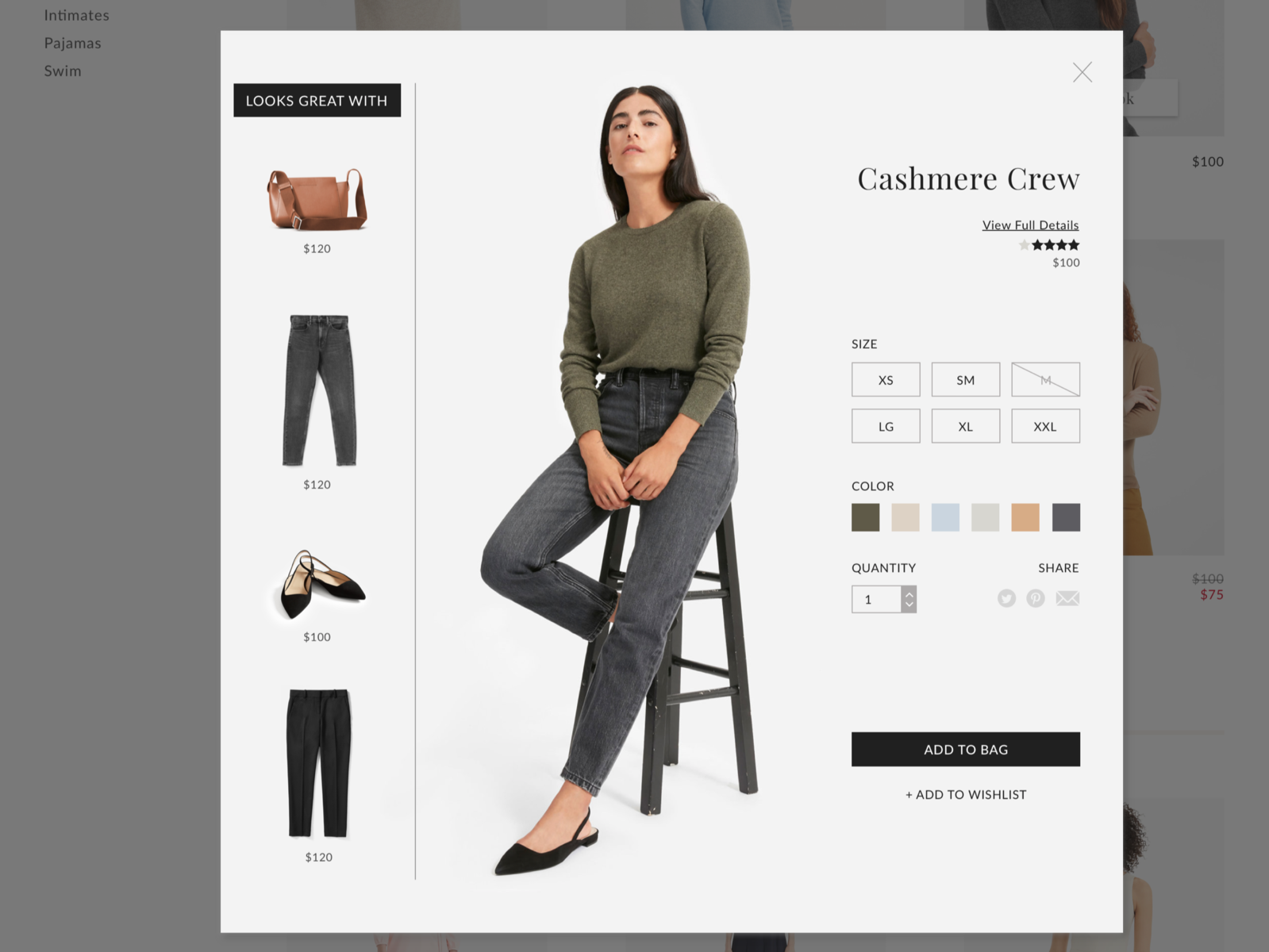In the image, a woman is seated on a stool, framed within a large white box. She has long, straight black hair cascading down her shoulders, with her chin slightly tilted upward, giving her a contemplative look. She is dressed in an olive green, long-sleeved shirt, and her hands are gently touching in front of her. She pairs the shirt with dark gray, skinny jeans that fit her form well, and finishes off her outfit with flat black shoes.

To the right of the woman, the text "Cashmere Crew" is prominently displayed. Beneath this title, the phrase "View Full Details" is underlined, inviting the viewer to learn more about the product. Below this, a rating system is shown with four black stars and one gray star, indicating a 4 out of 5-star rating. The price of the item is clearly marked with a dollar sign followed by "100."

Further down, the section for selecting the size is presented with squares labeled: XS (extra small), SM (small), M (medium, marked through), LG (large), XL (extra large), and XXL (double extra large). Below these size options, the word "Color" appears, with squares beside it illustrating the available colors: black, cream, blue, light gray, darker orange, and dark gray.

Lastly, the "Quantity" section is indicated by a box showing the number one. The image concludes with a black square containing the "Add to Bag" option, and a small plus sign beside the "Add to Wishlist" link, allowing the user to save the item for later.